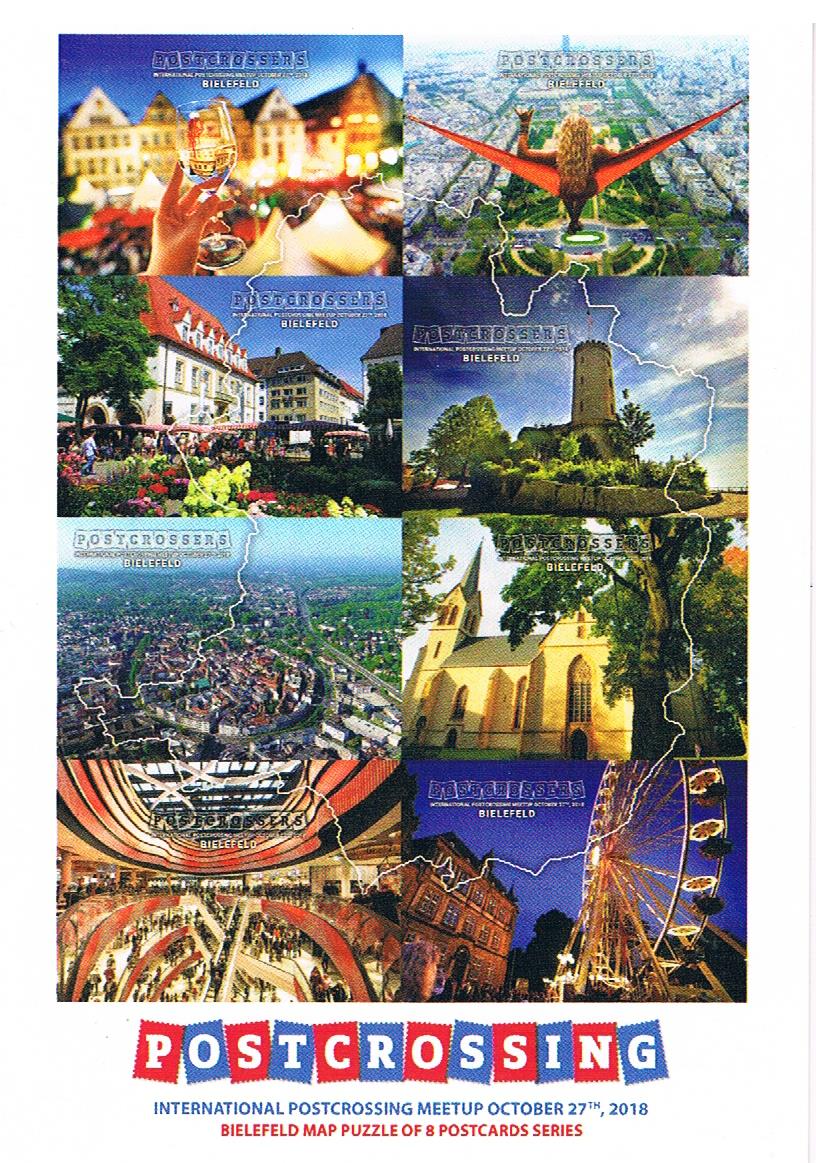This image features a collection of eight postcards, each depicting various landmarks and sights from a specific location, with an emphasis on Bielefeld. The postcards are arranged in two rows of four. 

Starting with the top row, the first postcard on the left showcases buildings that resemble a hotel and a hand holding a wine glass. Adjacent to it on the right, there's an aerial view of a city with numerous buildings, featuring a woman holding a glass, seemingly with wings. The middle two cards highlight a building with a red roof surrounded by vibrant flowers and shrubbery, while the last of the row displays part of a castle amidst green foliage.

The second row begins with another aerial perspective of a city. Next to it, there's what appears to be a cathedral or a church. Moving right, there's an indoor scene that may be an arena, convention center, or hotel. The final image shows a segment of a Ferris wheel and what could be a historical building.

Below the postcards, the text reads: "Post Crossing International Post Crossing Meetup October 27th, 2018 Bielefeld Map Puzzle of Eight Postcard Series." Each letter in the word "POSTCROSSING" is encased in a rectangular box resembling a stamp, alternating between blue and red. The date and event details are in blue uppercase text, while the series title is in smaller green uppercase letters.